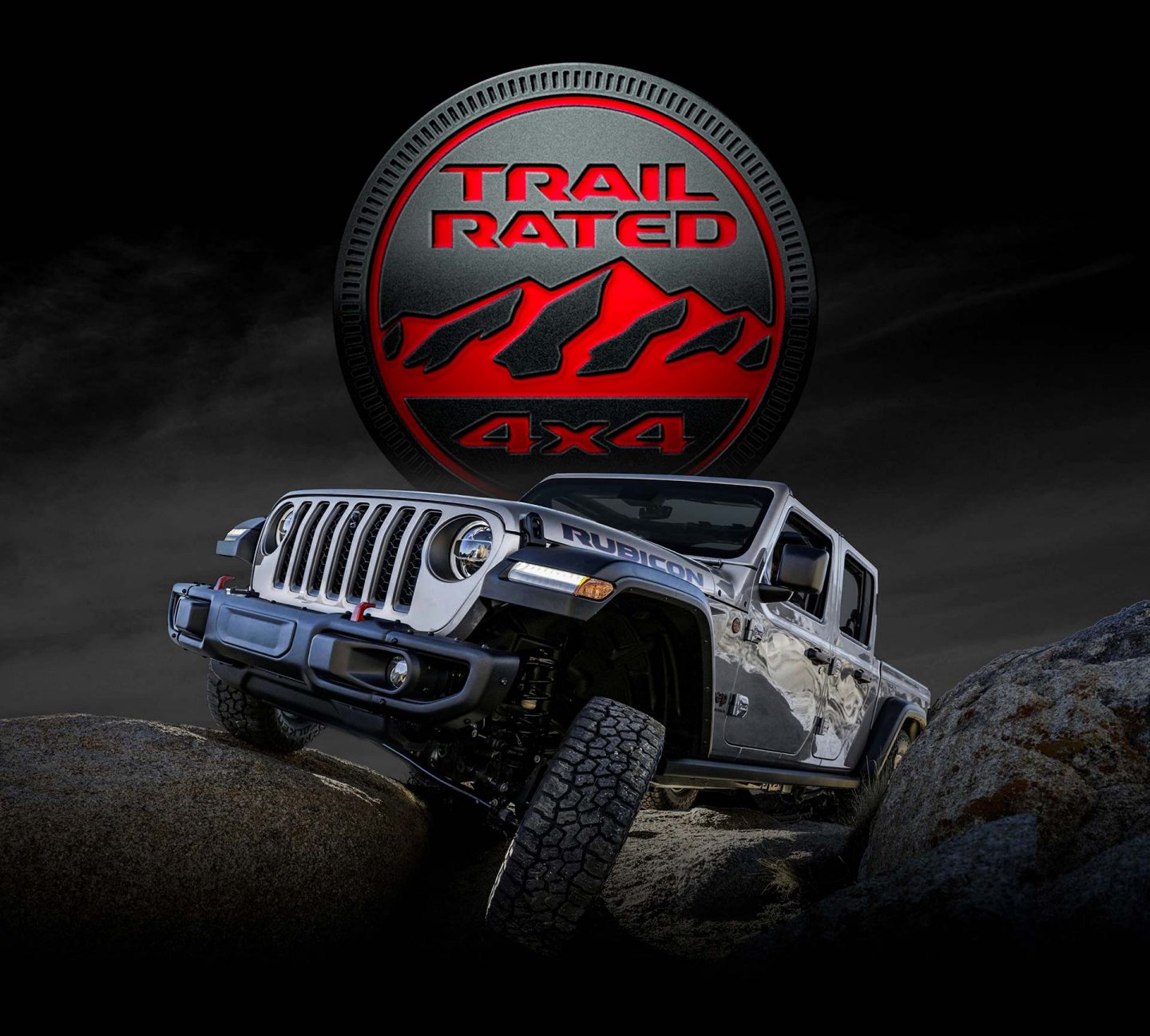The image features a rugged gray Jeep truck climbing over large, gray boulders, indicative of an off-road trail. The truck, labeled "Rubicon" in navy blue lettering on the side, showcases its power and capability with its front tire turned sideways as it navigates the challenging terrain. A prominent black circle with red accents on the vehicle bears the "Trail Rated 4x4" badge, featuring a red mountain range inside. The background combines ominous gray clouds and dark tones, highlighting the Jeep’s dominance in tough conditions.